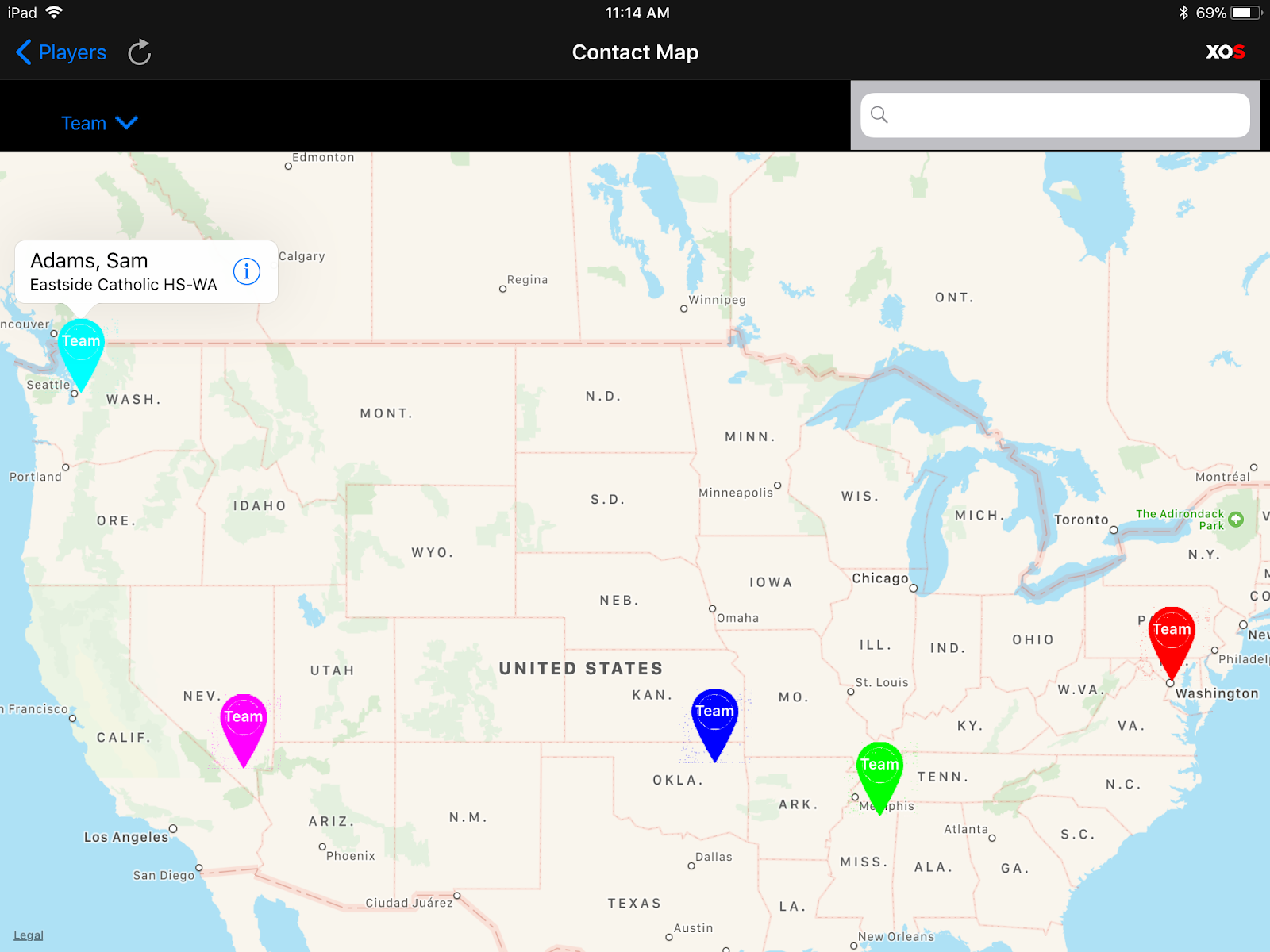The screenshot, taken from an iPad as indicated by the "iPad" label in the top left corner, captures a detailed view of a map-based application. The iPad is connected to Wi-Fi, shows a time of 11:14 AM, has Bluetooth enabled, and the battery is at 69%. The application displayed appears to be either a game or a tracking tool, featuring a "contact map" labeled as "XOS."

The primary interface reveals a menu with the option "Teams" selected. A highlighted entry reads "Adam Sam Eastside Catholic High School-WA." The map displays various teams marked with different colors across several states and regions: Washington (light blue), Nevada (pink), Oklahoma (blue), North Mississippi (green), and Washington D.C. (red). Each team is simply labeled as "Team," without specific names.

The map shown is of the United States and parts of Canada, although it excludes the southernmost areas of Texas and Florida. This detailed annotation of the teams and their locations provides a comprehensive snapshot of the application's current state.